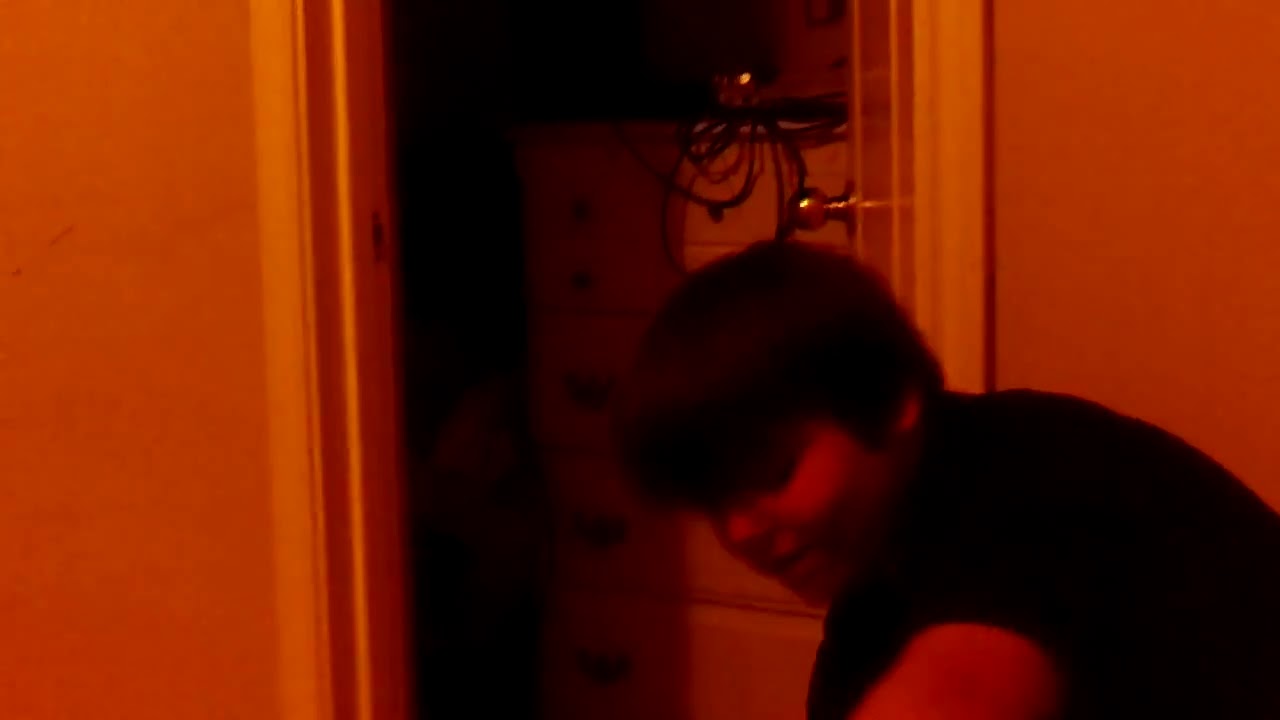In this low-resolution photograph, the entire scene is bathed in a yellowish-orange glow, likely due to a light source within the tan-colored room. In the lower right corner, a slightly chubby, younger individual with medium skin tone and short, dark brown hair is prominently featured. They are hunched over, their head lowered, partially obscuring their face. They're wearing a black short-sleeved t-shirt. The person's left ear is barely visible beneath their shaggy hair, and their partly open mouth adds to their slouched posture. Behind them, a white-framed open doorway reveals a white dresser adorned with some black cords draped across it. A shiny gold doorknob is visible above the individual, gleaming against the white doorway. The overall impression is one of a candid, possibly spontaneous photograph, characterized by graininess and compressed details, likely taken with a mobile phone.